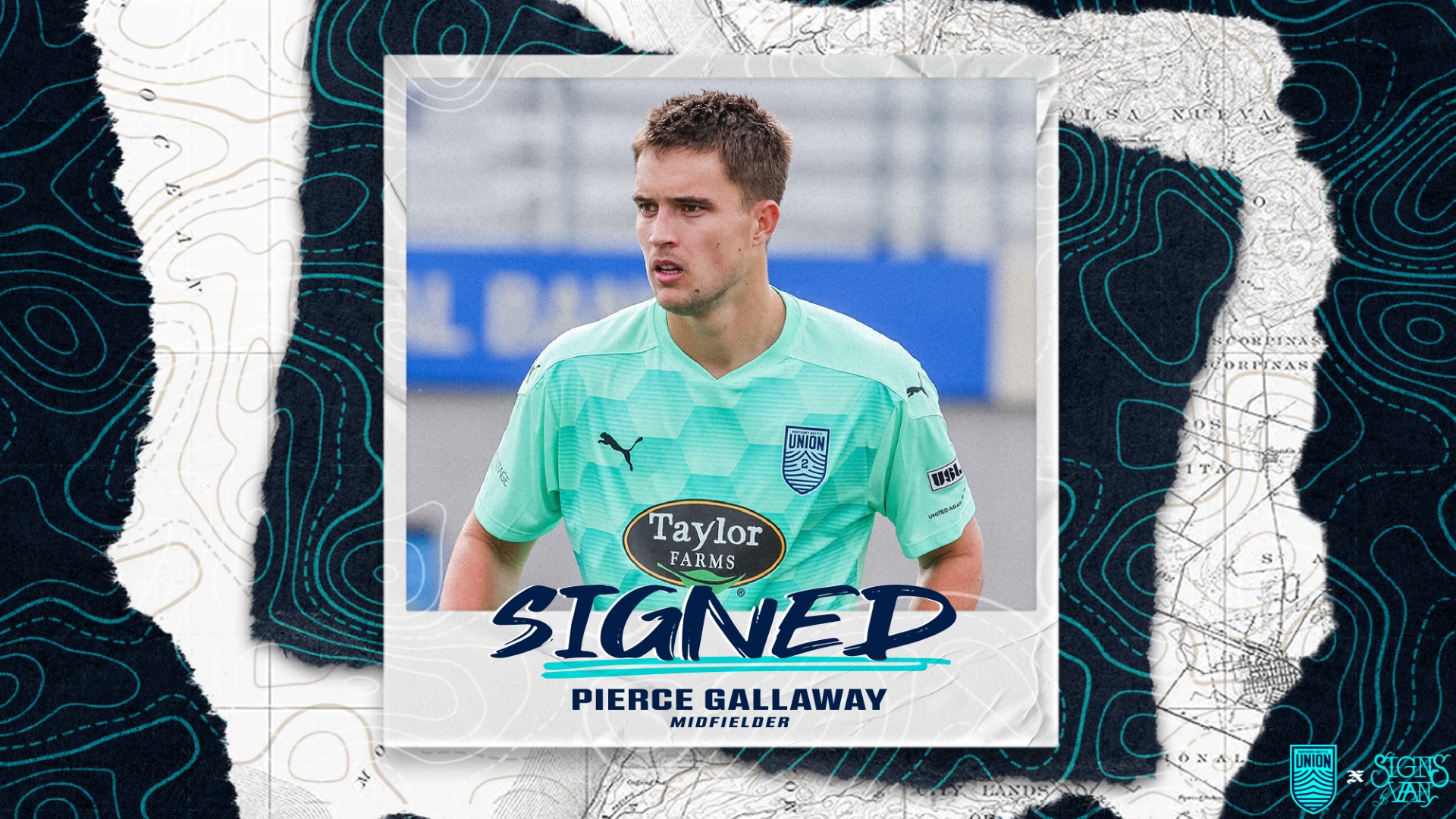This image is a color screenshot of an athlete named Pierce Galloway, who plays as a midfielder for a team sponsored by Taylor Farms. He is wearing a short-sleeved, teal athletic jersey adorned with a small jaguar emblem on the right breast, a shield-shaped team emblem on the left breast, and a central logo that reads "Taylor Farms." The athlete, a Caucasian male with short brown hair, is captured from the waist up, looking intently to the left with his mouth slightly open. The background is blurry, suggesting the edges of a stadium playing field, overlaid with what appears to be a blue and white abstract map of ocean currents or elevation levels. At the bottom of the image, there are two watermarks: one labeled "Union" and another that reads "Signs Van." The text underneath his picture states "Signed Pierce Galloway Midfielder," suggesting that this is a sports card or promotional material announcing his signing.